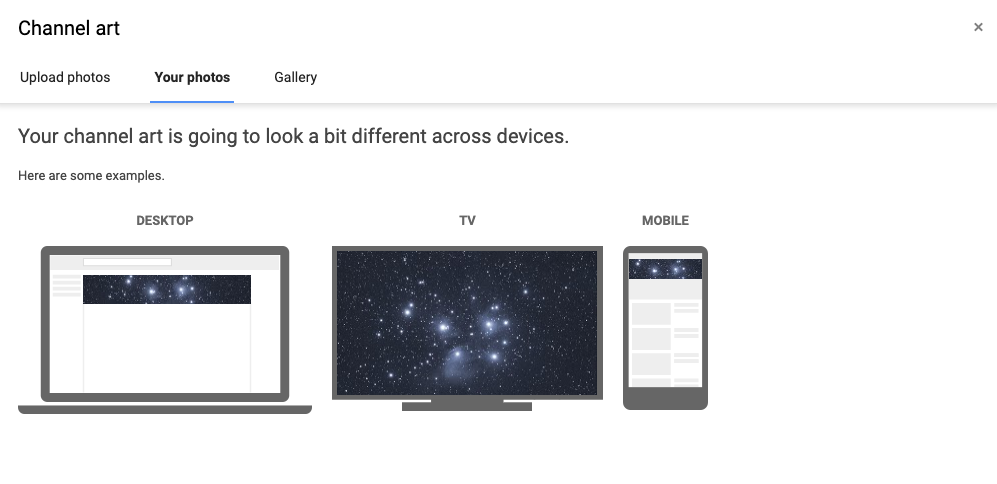The image showcases a webpage design with a minimalist white background and black text. At the top left corner of the webpage is the title "Channel Art." Below this heading are three organized sections: "Upload Photos," "Your Photos," and "Gallery." The section "Your Photos" is currently highlighted, indicated by a blue horizontal line underneath it. Beneath this, a message in black text reads, "Your Channel Art is going to look a bit different across devices." Below that, in smaller black text, it says, "Here are some examples."

Three examples follow, demonstrating how the channel art will appear on different devices: desktop, TV, and mobile. 

1. **Desktop View:** Depicted as a laptop with a dark gray bezel around the screen, which is open to a white webpage. The banner on this page features stars against a black background.
  
2. **TV View:** Shown as a flat-screen TV with a gray bezel, mounted on a stand. The TV screen displays a dark background with illuminated stars, representing a space scene.

3. **Mobile View:** Illustrated as a smartphone resembling an iPhone, with a dark gray highlighted bar. The screen shows a similar webpage with a white background and a space-themed banner featuring dark skies and stars.

Overall, the image effectively demonstrates the visual consistency of the channel art across different device interfaces while highlighting their unique display attributes.